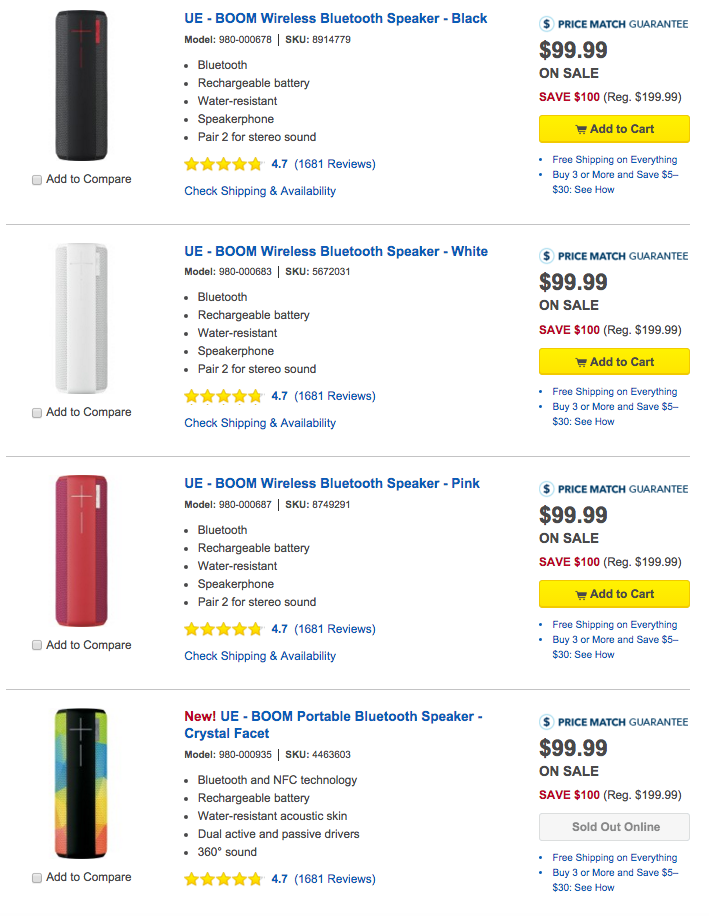This vertical image appears to be a product comparison from Amazon that you can access via a smart device or computer. The background of the image is plain white, likely using the default white screen color of the user's computer. 

The image is a detailed comparison of different wireless speakers, each represented by an icon of the speaker, the name, and essential information including the price and purchasing options. 

1. **Black Speaker**:
   - **Name**: UE Boom Wireless Speaker in Black
   - **Details**: Model number provided, supports Bluetooth, rechargeable battery, water-resistant, speakerphone capabilities, and stereo sound pairing.
   - **Ratings**: 4.7 stars based on 1681 reviews.
   - **Price**: Originally $199.99, now on sale for $99.99, saving $100.
   - **Additional Info**: Price match guarantee, free shipping, option to check shipping availability, and a promotion to save $5 to $30 when purchasing three or more.

2. **White Speaker**:
   - **Name**: UE Boom Wireless Speaker in White
   - **Details**: Identical to the Black version including Bluetooth, rechargeable battery, water-resistant, speakerphone capabilities, and stereo sound pairing.
   - **Ratings**: Holds the same 4.7 stars from 1681 reviews.
   - **Price**: Same pricing and discounts as the Black version - $99.99 on sale from the original $199.99.
   - **Additional Info**: Includes all mentioned promotions and shipping options.

3. **Pink Speaker**:
   - **Name**: UE Boom Wireless Speaker in Pink
   - **Details**: Consistent with Black and White versions - Bluetooth, rechargeable battery, water-resistant, speakerphone capabilities, and stereo sound pairing.
   - **Ratings**: Maintains the 4.7-star rating from 1681 reviews.
   - **Price**: Identical - $99.99 on sale from the original $199.99.
   - **Additional Info**: Same promotional offers and shipping details as the previous colors.

4. **Crystal Facet Speaker**:
   - **Name**: UE Boom Portable Bluetooth Speaker in Crystal Facet
   - **Details**: Similar features to the other models including Bluetooth capability, rechargeable battery, water resistance, speakerphone, and stereo sound pairing.
   - **Ratings**: Not specified, inferred similar high rating.
   - **Price**: Matches the sale price of $99.99 from a regular price of $199.99.
   - **Additional Info**: Promotion details and shipping options similar to the other models.

Each speaker can be added to the cart directly from the image interface, with options to check shipping availability and details on the price match guarantee.